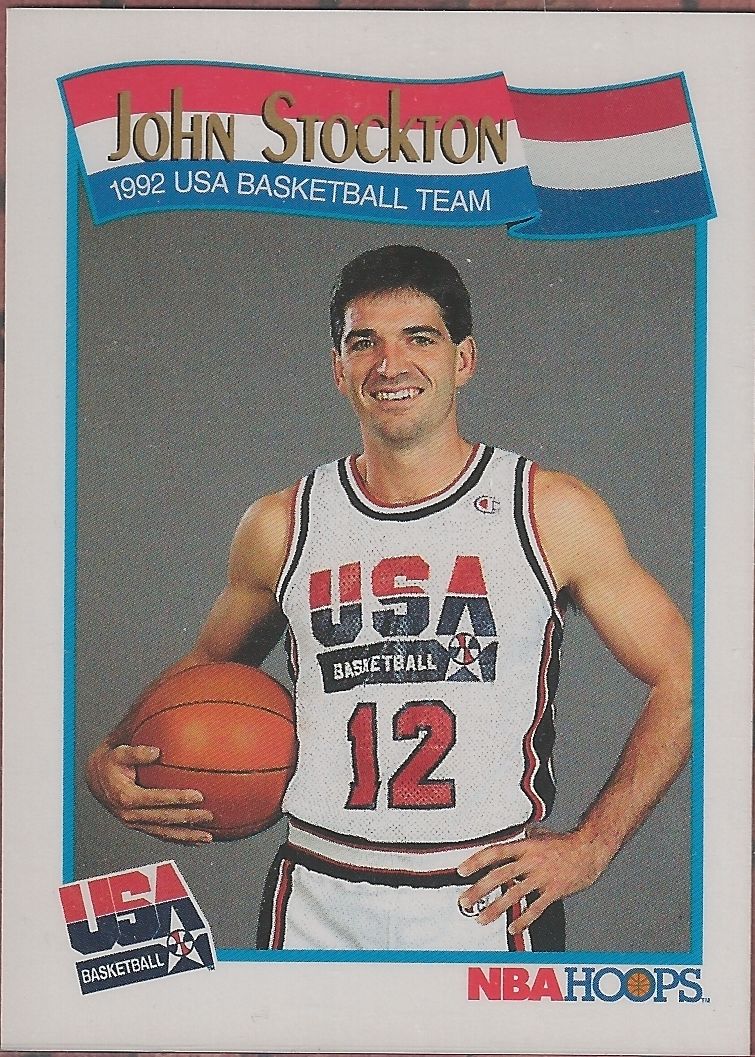The image is a classic 1992 basketball card featuring John Stockton from the USA basketball team. At the very top of the card, in golden-yellow text, it reads "John Stockton" across a red, white, and blue banner. Below that, in white text, it states "1992 USA Basketball Team." The central image shows John Stockton with short, thick black hair and a smiling face, revealing his top teeth. He is wearing a white jersey with "USA" on the chest, where the top half of "USA" is red and the bottom half is blackish-blue. Beneath "USA," there's a black bar with the word "Basketball" in white text, followed by the player number "12" in red text.

The basketball is held between Stockton's right arm and his stomach, with his left hand grabbing his wrist. On the left side of the card, there's another "USA Basketball" inscription with a star icon. At the bottom right corner, "NBA Hoops" is written in red and blue text, with the second "O" replaced by a basketball icon. The card brings back memories of 90s basketball memorabilia, and it was a valued piece in many collections.